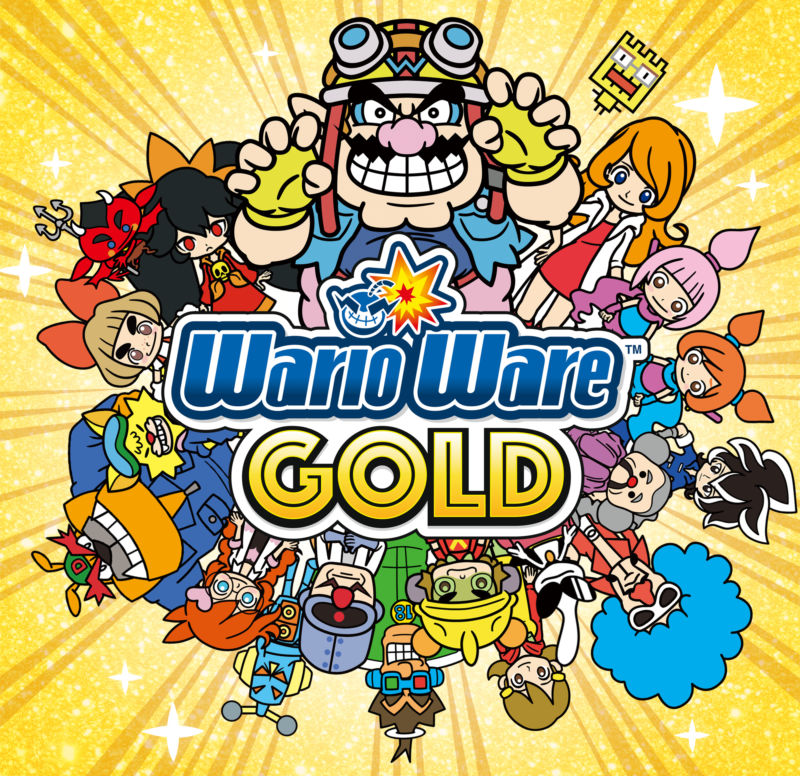The image is a square cartoon advertisement for "WarioWare Gold." The background is a golden color, dotted with white stars that appear to be lit up, giving a glowing effect. At the center is the title "WarioWare Gold." "WarioWare" is written in blue bubble letters outlined in white, while "GOLD" is encapsulated in gold letters, outlined in black against a white backdrop.

Above the title, prominently featured, is the character Wario from the Super Mario universe. He has a menacing expression with his teeth bared and hands posed like claws. Wario sports a pink nose, a hat with a large "W" in the center, and goggles resting on his head. He has a distinctive black mustache.

Surrounding Wario and the title are about 20 smaller cartoon characters arranged in a circular pattern. These characters seem to be part of Wario's universe, each with unique and colorful designs - ranging from children to quirky, cool personalities, and even a blue-haired disco dancer. The character designs are diverse, featuring a variety of colors, including blue, orange, yellow, brown, white, and purple. Notably, one character wears a skull necklace and has red eyes, adding to the eclectic mix. The background complements the lively scene with a starburst pattern, radiating lines from the center, enhancing the overall dynamic and vibrant appearance.